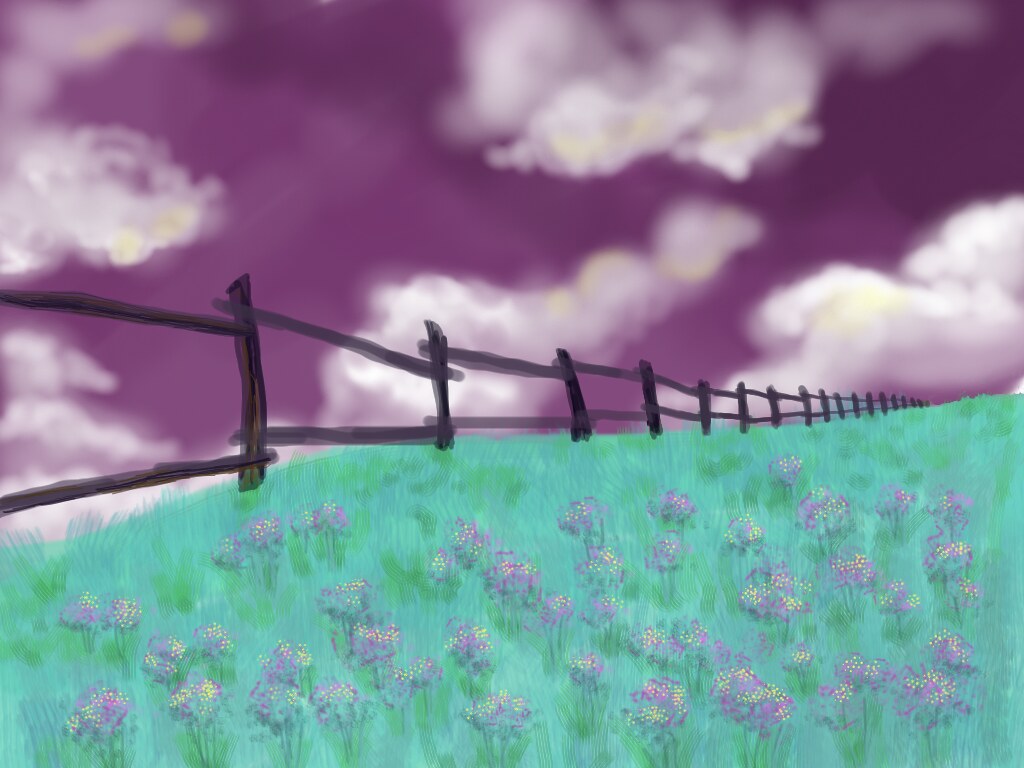This illustration, seemingly a blend of digital techniques and traditional pastel aesthetics, showcases a serene evening scene. The upper half features a dreamy purple sky adorned with both sharply-focused white clouds and wispy, ethereal formations, capturing the transient nature of cloudscapes. Below, a verdant hillside emerges, bathed in hues of blue-green, almost aqua, grass. Amongst this sea of color, clusters of green-leaved plants grace the landscape, each topped with vibrant purple flowers. These blooms, characterized by their rounded clusters and delicate yellow or white specks, stand out distinctly, hinting at the meticulous detail captured in each petal. Anchoring this pastoral scene, a split rail fence stretches diagonally from the left foreground to the distant right, guiding the viewer's eye towards the softly fading horizon. This fusion of natural elements and artistic approach evokes a tranquil, almost otherworldly, rural paradise.